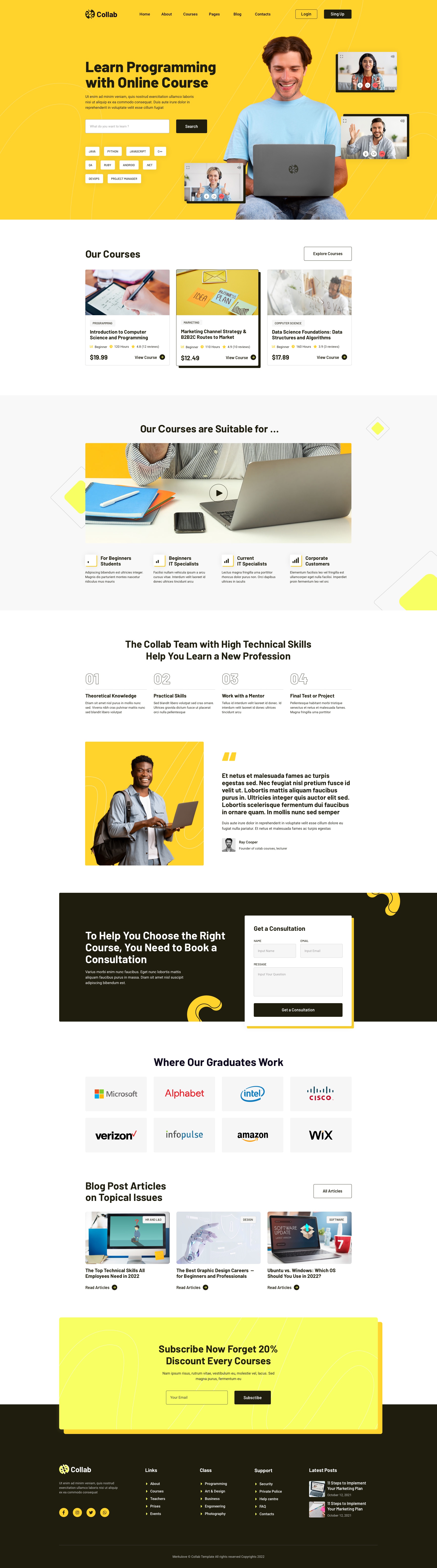This image is a screenshot of a web page featuring an online learning platform. The layout appears slightly distorted, with both text and images stretched, giving the page a wider appearance and causing some elements to appear slightly warped.

The top bar of the page is highlighted in yellow. In this bar, on the left-hand side, the website's logo reads "Collab" in black text, accompanied by menu options like Home, About, Courses, Pages, Blog, and Contacts, as well as buttons for logging in and signing up.

Below the top bar, a main feature displays a cheerful image of a man with brown hair, smiling as he sits at a laptop. He's dressed in a blue shirt and blue jeans. On his laptop screen, three separate video feeds show other individuals engaged in what appears to be a Zoom conference call; they are smiling and waving at the viewer.

To the left of this central image, there is a prominent heading that reads "Learn Programming with Online Courses." Below this heading, there is a search input box accompanied by a black search button, encouraging users to look for specific courses.

Further down the page, the section labeled "Our Courses" showcases several options available to users. Featured courses include "Introduction to Computer Science and Programming" priced at $19.99, and "Marketing Channel Strategy and B2B to C Routes to Market" priced at $12.49.

Additional information highlights that the courses are suitable for beginning students, beginner IT specialists, and corporate customers. There is also an image of a man with a backpack, holding a laptop in front of him, reinforcing the theme of mobile and accessible learning.